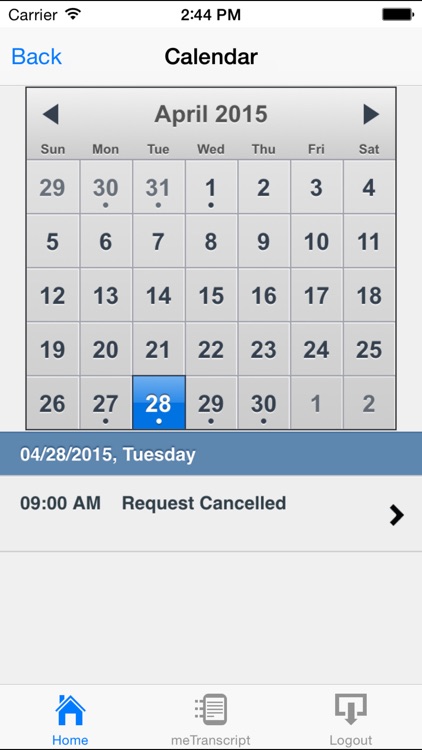In this image, we see a calendar page set against a dark background, displaying the month of April for the year 2015. The date, Tuesday, April 28th, is prominently highlighted. The calendar is formatted with the days of the week running from Sunday to Saturday. 

At the top of the image, there are several icons: Home, Me, Transcripts, and Logout. These icons are also duplicated at the bottom of the image. In the calendar's notes, there is an entry that reads "SmarterText, 9am, request cancelled," specifically referring to the highlighted date of Tuesday, April 28th, 2015. 

The image effectively communicates the details of the specific date and the scheduling note associated with it, while also providing user interface icons for navigation within the application or platform depicted.